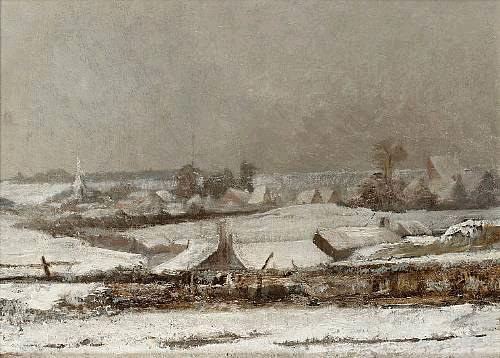This artwork, likely a painting, captures a serene yet somber winter scene of an old European village, possibly from the 1800s. Dominated by grays, browns, and whites, the sky takes on a grayish, stormy hue, complementing the snow-covered landscape below. In the foreground, weathered huts or farm structures, seemingly made of wood and straw, show signs of activity with paths worn into the snow. Sparse, leafless trees are scattered around, adding to the barren atmosphere. 

Further back, a collection of rooftops and buildings, intentionally blurred for depth, extends into the distance, suggesting a small town blanketed by snow. These structures, characterized by tall, A-frame roofs designed to manage heavy snowfall, hint at the region's harsh winters. The scene suggests a remote farm or village with no visible signs of life—no animals or people—emphasizing the quiet stillness of the season. A barbed wire fence along what appears to be a road adds to the rustic, tranquil, and slightly desolate feel of this winter depiction.